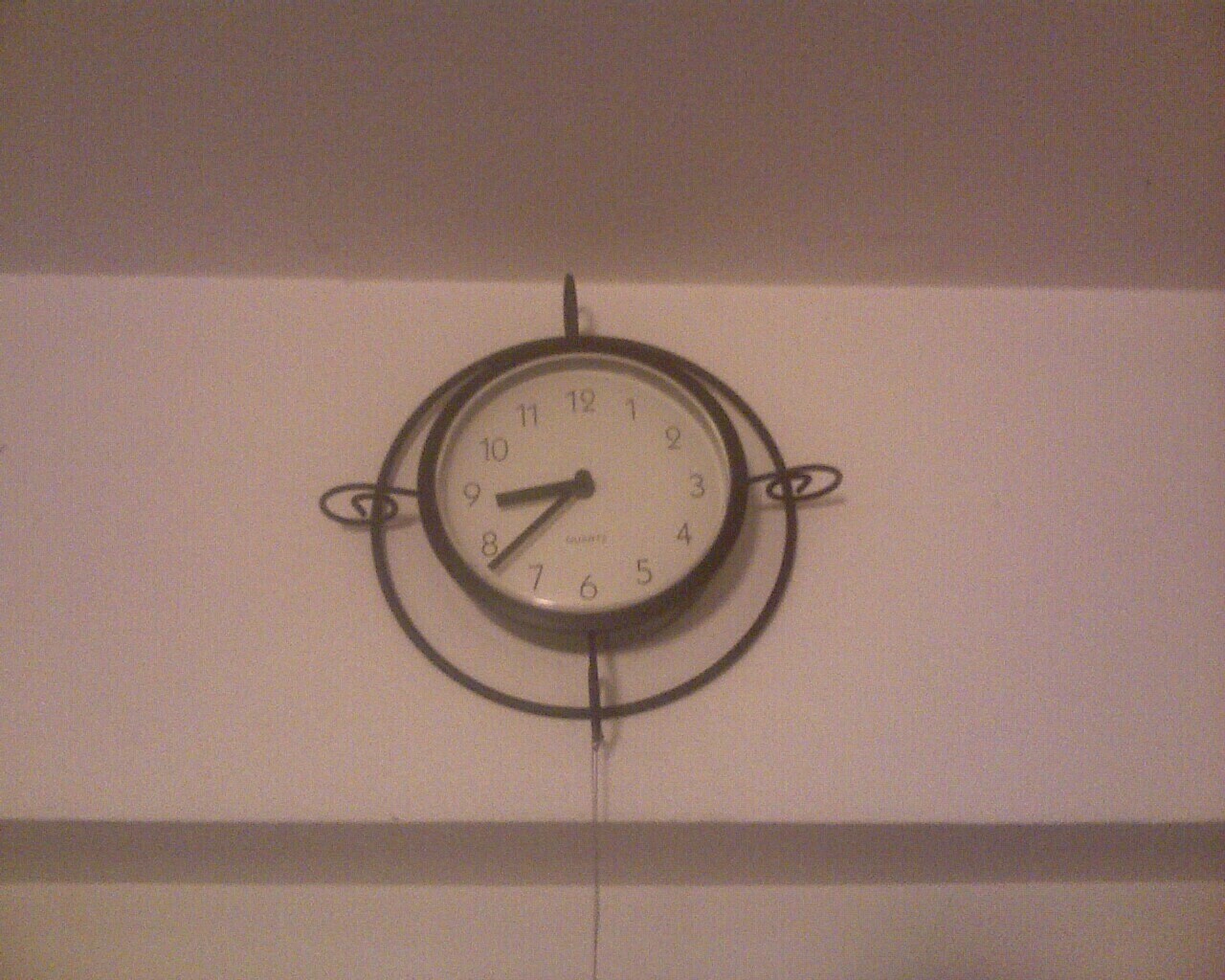The image captures a distinctive wall clock, potentially located in a kitchen or classroom, mounted on a soffit. The clock is encircled by an ornate iron ring, adorned with scrollwork extensions at the 12, 3, 6, and 9 o'clock positions, creating an intricate, perpendicular design element against the main circular frame. The clock itself features a classic black border, a stark white face with standard Arabic numerals, and black clock hands indicating the time as approximately 8:40. The word "quartz" is inscribed at the bottom of the clock face, with no other identifying markings visible.